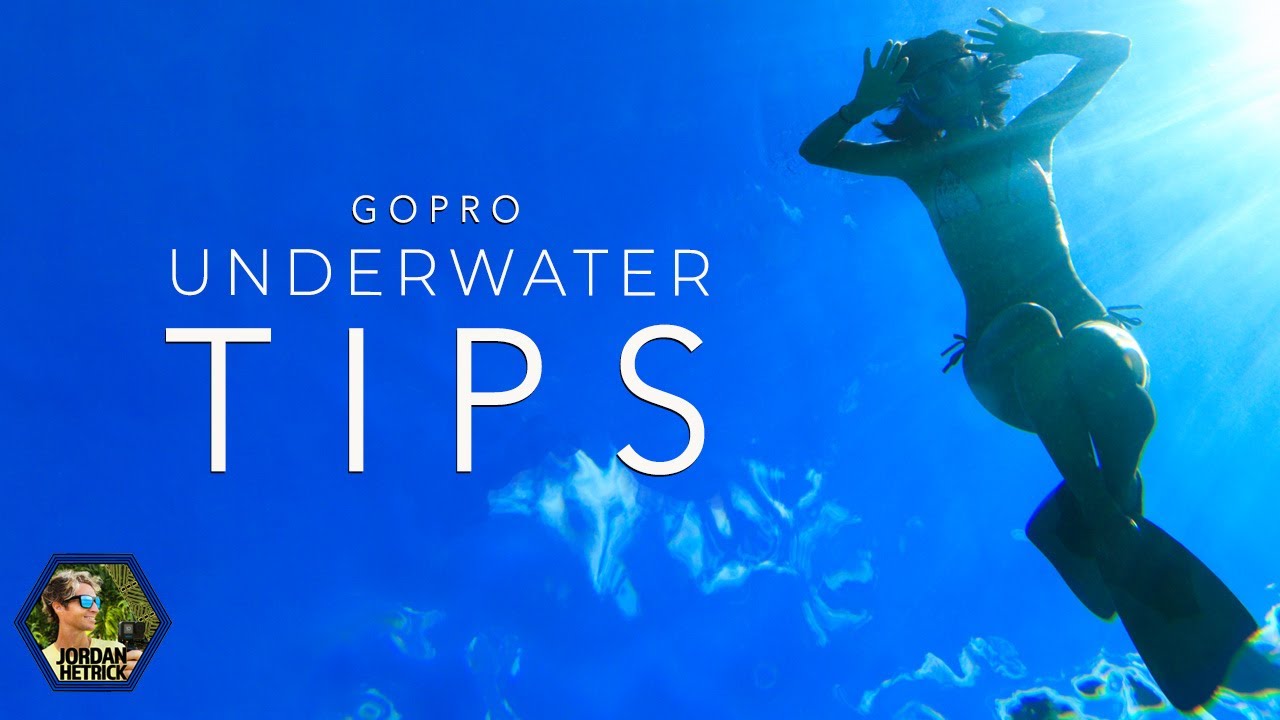The image is an advertisement for GoPro Underwater Tips, featuring an instructional guide on using the GoPro for underwater activities. The scene captures the perspective from beneath the water's surface, looking up at a woman in a swimsuit with a snorkel mask and fins. She appears to be floating with her hands up and her legs crossed, gazing into the distance. The water around her is a deep blue with artistic light blue accents and sun rays piercing through the surface in the upper right corner. Bold white text to the left reads “GoPro Underwater Tips,” emphasizing the focus on underwater photography guidance. In the bottom left corner, there's a solid frame with the name and picture of Jordan Hetrick, who is likely the creator or the instructor associated with the content.